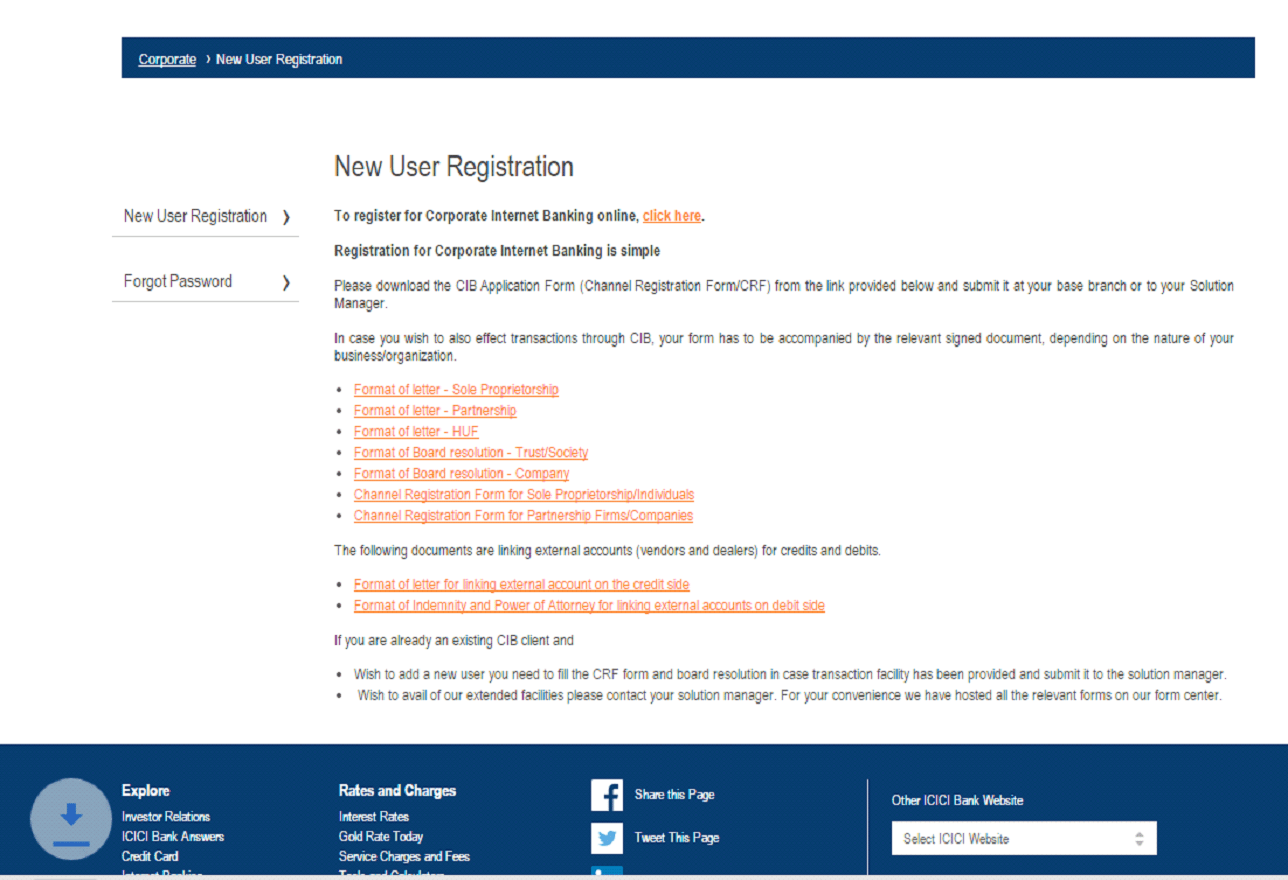**Detailed Caption for the Image**

The image is a screenshot taken from a corporate internet banking website. At the top, there's a dark blue bar spanning across the width of the screen with white text, indicating the website's title and available options.

### Top Navigation Bar:
- **Corporate**
- **New User Registration**

### Main Content Area:
Set against a clean white background, there's a detailed panel laid out with instructions and essential information on the left half of the screen.

#### Left Column:
- **New User Registration**
- **Forgot Password**

#### Right Column:
A comprehensive guide on registering for corporate internet banking is provided:

1. **New User Registration**:
   - **Click here** (highlighted in orange) for corporate internet banking registration.
   - The process is described as simple. It instructs users to download the CIB (Corporate Internet Banking) application form from the provided link, and submit it at their base branch or to their solution manager.
   - Users wishing to perform transactions through CIB must include the relevant signed documents, depending on their business or organization type.

2. **Required Documentation**:
   - This section lists various documents needed for registration, presented as clickable links (highlighted in orange), which lead to specific form templates:
     - **Format of Letter – Sole Proprietorship**
     - **Format of Letter – Partnership**
     - **Format of Letter – HUF (Hindu Undivided Family)**
     - **Format of Board Resolution – Trust/Society**
     - **Format of Board Resolution – Company**
     - **Channel Registration Form for Sole Proprietorship/Individuals**
     - **Channel Registration Form for Partnership Firms/Companies**

3. **Linking External Accounts**:
   - Additional documents for linking external accounts with credits and debits are also provided as links in orange:
     - **Format of Letter for Linking External Accounts – Credit Side**
     - **Format of Indemnity and Power of Attorney for Linking External Accounts – Debit Side**

4. **Existing CIB Clients**:
   - Instructions for existing CIB clients who wish to add a new user:
     Require filling out a CRF (Customer Relationship Form) and a Board Resolution, and submitting it to their solution manager.
   - Contact details for availing extended facilities are also provided, encouraging clients to reach out to their solution manager.
   - A note about the availability of all relevant forms at the form center for user convenience.

### Bottom Navigation Bar:
Lastly, a dark blue bar at the bottom of the page offers quick links for further exploration:
- **Explore**
- **Rules and Charges**
- **Facebook Share This Page**
- **Tweet This Page**
- **Other ICICI Bank Websites**
- **A Pull-Down Menu** for additional options

This structured and detailed layout facilitates ease of navigation and ensures that users can efficiently access the information and documents they need for corporate internet banking registration and related activities.